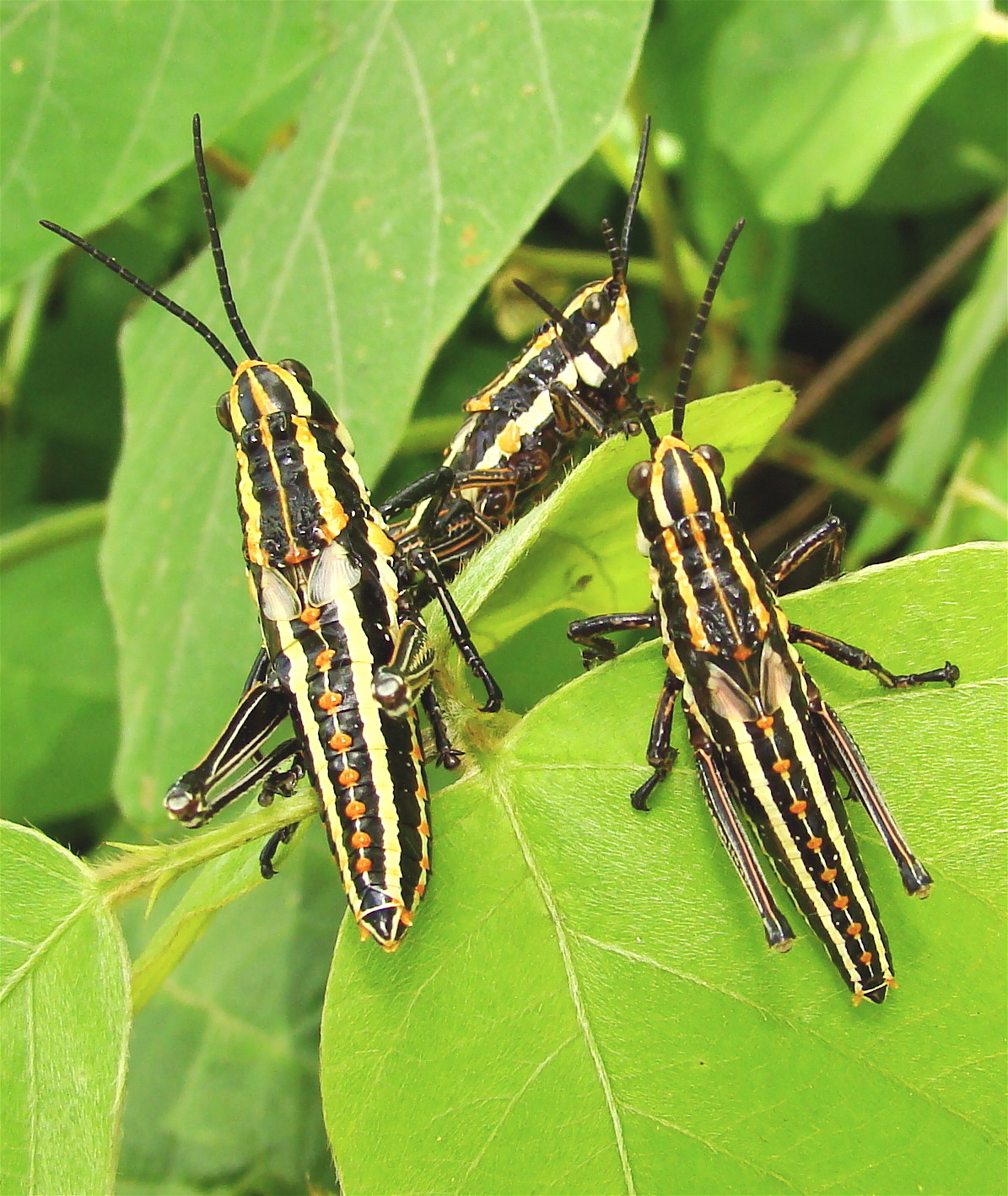This highly detailed close-up photograph captures three distinct insects, resembling grasshoppers or potentially praying mantises, perched on a cluster of five lush green leaves. Each insect, approximately two inches in length, is characterized by striking black and yellow stripes along its elongated body. They boast six legs, with four firmly gripping the leaves and the hindmost pair positioned for potential jumping. Their appearance is further accentuated by prominent black eyes and two black antennae protruding from their heads. The focus of this clear, professionally-shot image centers on these three insects, meticulously showcasing their unique features and interactions with the leaves. This image serves as an intriguing visual study of these insects in their natural environment and could be ideal for educational material or an entomology website.